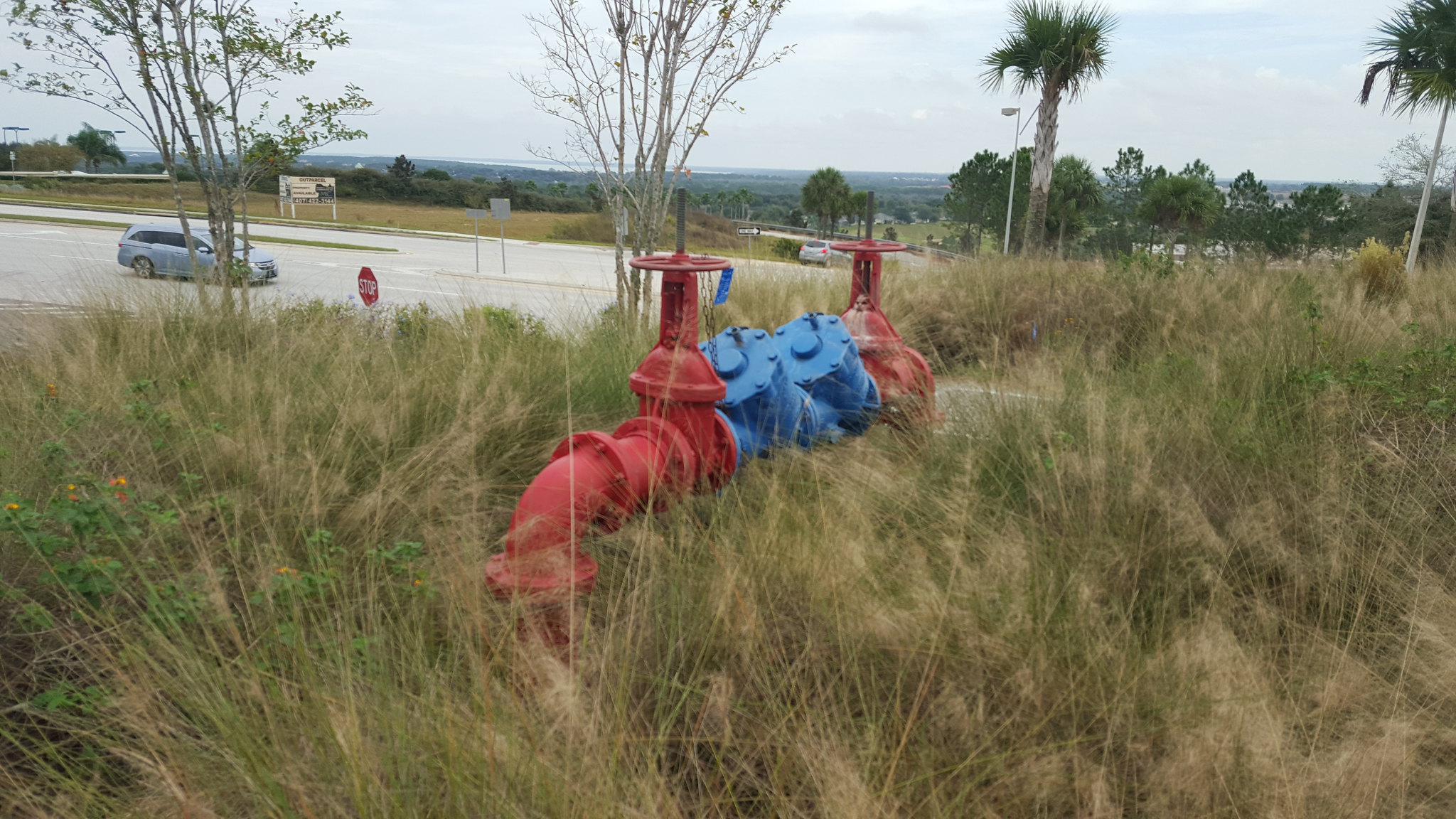The photograph, taken outdoors, captures a scene dominated by a cloudy, gray sky stretching towards a distant horizon. The area is rich with vegetation, including a variety of trees—some recognizable as palm trees with thick brown trunks and pointy green leaves, others more indistinct. A highway featuring a divider, a guardrail, and a minivan is visible, alongside a parking lot that hosts a single light blue van. Prominently in the foreground, a field of tall, thick, and overgrown green grass is interspersed with small yellow flowers. Nestled within this grassy area, there is a distinctive red and blue metal structure, possibly a fire hydrant or a meter, with red valves and blue piping, indicating two sections. A stop sign marks the scene, adding to the sense of human presence within this lush and varied environment.